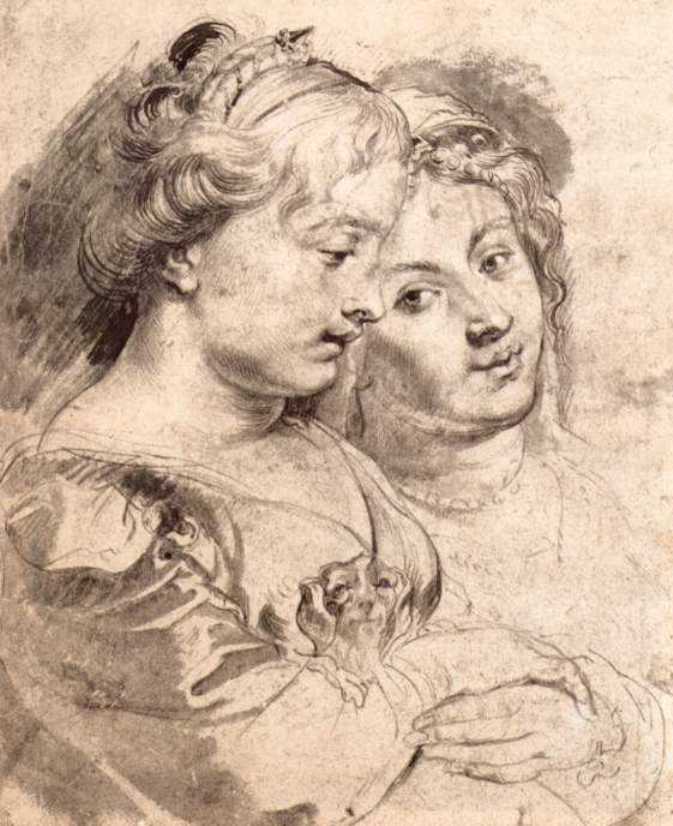This vertical rectangular image is a sepia-toned sketch, possibly done with pencil or charcoal, depicting two women in an embrace. Both women, facing toward the right, have long, curly hair. The woman on the right, seen in full face, has small tendrils of curls framing her face, while the woman on the left, seen in profile, has her hair styled in barrel rolls around her face and neck. They both exhibit fair skin and light hair, likely blonde, given the lack of shading. Their outfits appear ornate and historical, reminiscent of 1800s fashion, with v-cut tops and flouncy sleeves. The woman on the right is adorned with a necklace, and the woman on the left, dressed in a low-cut, heavy velvet-like dress, is holding a small dog with floppy ears and a fuzzy tail. The sketch is detailed mainly around their faces, highlighting their light eyebrows, cupid's bow lips, and chubby cheeks. The background remains white, emphasizing the meticulous portrayal of their tender moment.